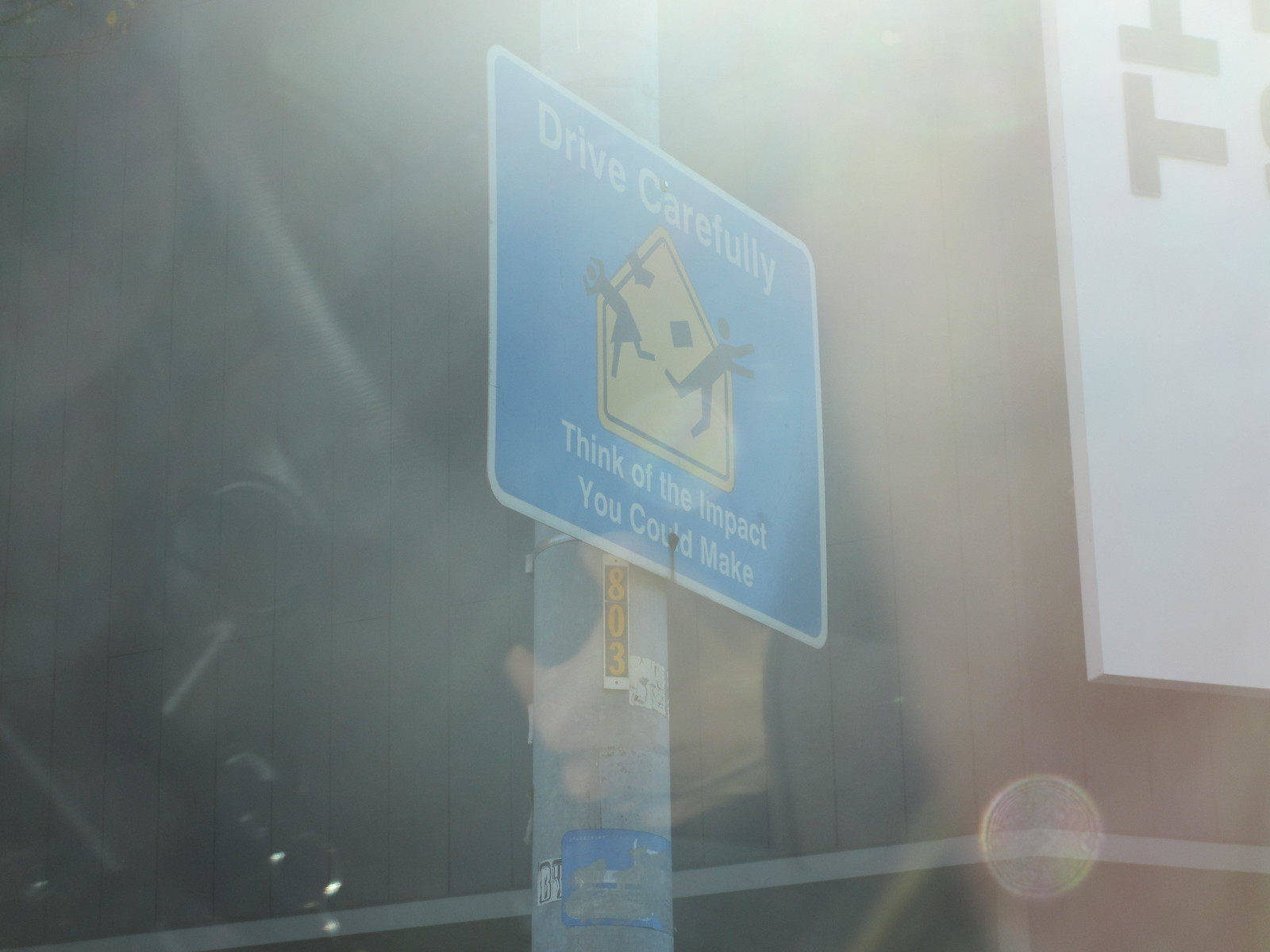This outdoor color photo is taken through a windshield or window, making the image appear very hazy and semi-blurry. The sunlight casts orb-like spots in the bottom corner, adding to the washed-out effect. At the center of the photo, there is a blue sign with white trim. Written in white letters on the sign are the words: “Drive carefully. Think of the impact you could make.” Below these words, there is a caution yellow image showing two stick figure-like characters depicted as falling, adding a visual element to the warning. This image uses a play on words to emphasize the importance of driving safely, with "impact" referring both to the physical consequence of a car accident and the positive effect of careful driving. To the right, partially out of frame, there is another white sign with the letters "TH" visible. The light background and overlay of dark and bright elements create a hazy yet vivid reminder to drivers.